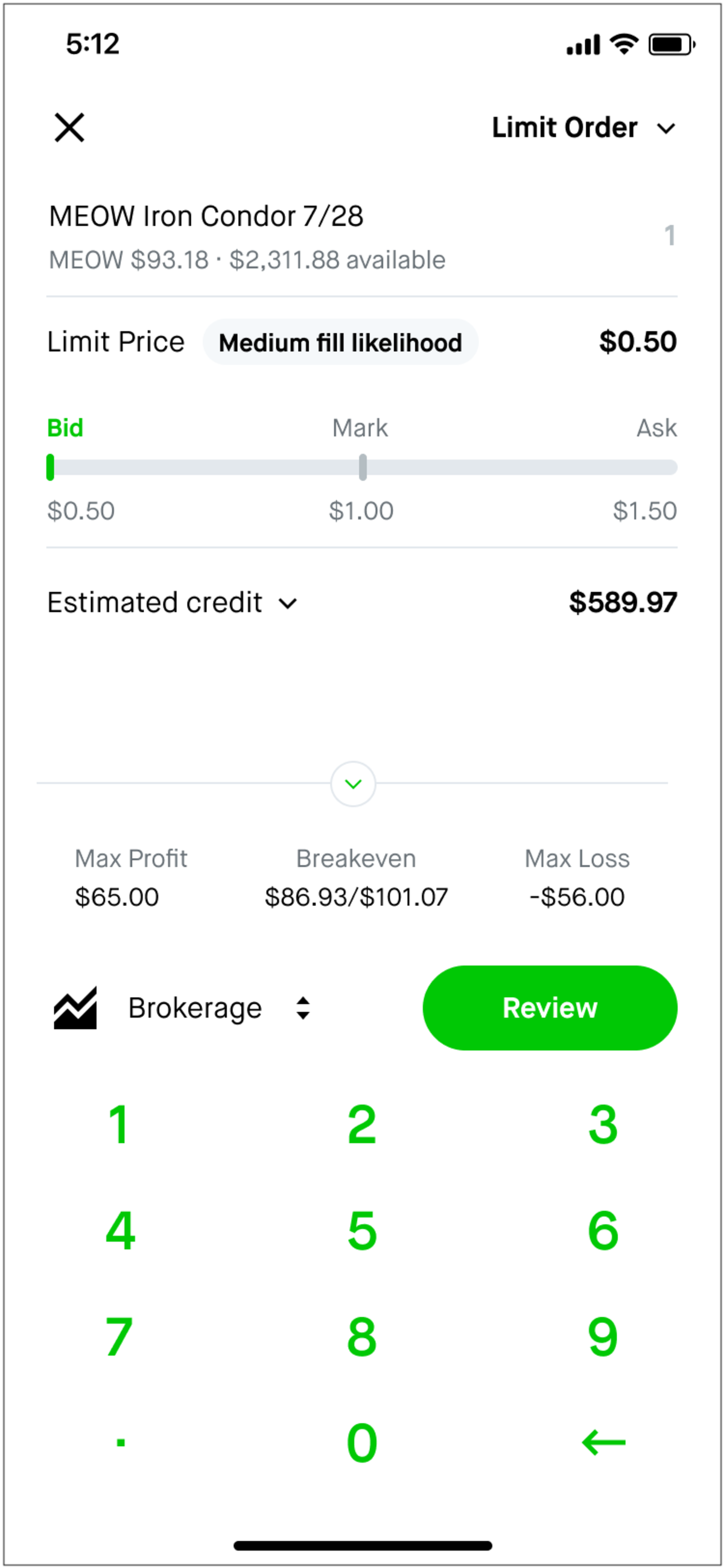This image, likely a screenshot from a mobile device, displays a detailed brokerage review interface. At the top of the image, the status bar shows the time (5:12), along with icons indicating internet service, phone connectivity, and battery level. Directly below, on the right side, there is an option labeled "Limit Order."

The left side features a stock option titled "Meow Iron Condor 728," followed by relevant details "Meow 933.18.2311.88," indicating available funds. Below this, "Limit Price" and "Medium Fill Likelihood" are centered on the screen, with "50 cents" listed to the right.

The interface provides different price options: "Bid" at $0.50, "Mark" at $1.00, and "Ask" at $1.50. The estimated credited amount is displayed as $589.97, unexpanded from a dropdown menu.

Further down, it shows potential financial outcomes:
- Max Profit: $65
- Break Even: $86.93 / $101.07
- Max Loss: -$56

A "Brokerage" section includes a button for reviewing brokerage details. The bottom section of the image features a green numerical keypad with the numbers 1 through 9, 0, a dot, and an arrow, set against a predominantly white background.